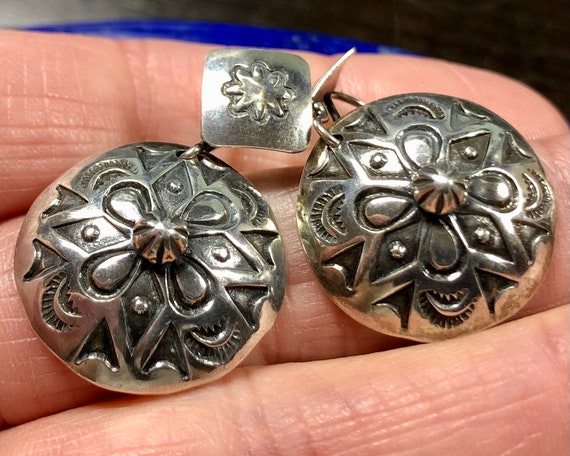The image is a sharply focused, photorealistic, color photograph in landscape orientation, depicting a pair of intricate silver earrings resting on the upturned fingertips of a person's hand. The fingers, extending from the left side of the image, are showcased from the joints to the fingertips, revealing the fine lines and fingerprints, indicating the closeness of the shot. The background is black, ensuring that full attention is drawn to the highly detailed earrings.

Each earring features a central design built around two large, connected circles. Within the inner raised circle is a flower-like pattern with four petals radiating from the center, surrounded by triangular and diamond-shaped engravings that resemble leaves. This mandala-style decoration extends outward to form complex, decorative motifs.

At the top of each earring, a square piece, set with one corner facing downwards, connects to the circular body. This square piece has an elaborate star or flower-like design at its center, enhancing the earring's ornate appearance. The photograph illuminates the earrings' silver tones with hints of gray and black to accentuate the depth and detail of the engravings. The overall style of the image emphasizes photographic representational realism, capturing every minute detail with clarity.